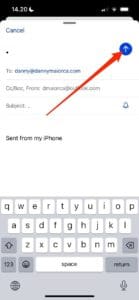The image is a screenshot from a smartphone, showing a search result page against a black border at the top. The time displayed is 14:20, accompanied by a small half-moon icon, indicating that Do Not Disturb mode is active. On the top right corner, the screen shows the remaining battery life and the signal strength bars. Below these details, there is a "Cancel" button. The image is somewhat blurry, making the specific search result difficult to read. However, a bold red arrow, angled diagonally upward across the search result, points towards a round blue button with a white arrow inside, suggesting a recent action or emphasis on this part of the screen. The phrase "Sent from my iPhone" is visible, indicating that the screenshot might be from an email or a messaging app. At the bottom of the image, there's a prominently displayed QWERTY keyboard, with keys highlighted in white and dark letters. The first row of letters starts with Q-W-E-R-T-Y-U-I-O-P, while the last row includes Z-X-C-V-B-N-M. Additional keys such as the backspace icon, return button, upward arrow, numeric "1-2-3" button, and a small microphone icon are also visible, commonly used for typing and voice input functions on a smartphone.